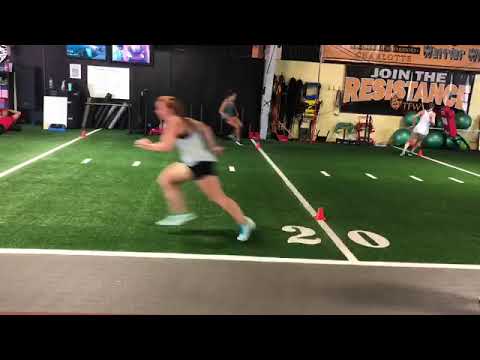The image depicts an indoor sports practice field that closely resembles an outdoor American football field. The field is vibrant green with distinct white lines, including a clear marking for the 20-yard line and smaller white bars splitting the field. Prominent on the field is a woman sprinting energetically to the left side of the image, her motion captured in a blur. She has reddish-orange hair tied back and is dressed in a light blue tank top, which partially reveals a black sports bra underneath, black shorts, and turquoise shoes. In the background, other women are engaged in various athletic activities, including one seated and another training with a ball. The far wall of the indoor facility is adorned with several posters, one notably bearing the words "Join the Resistance." Around this area, there are various items scattered, including large green balls. Additionally, a banner reading "Charlotte Warrior" is visible, contributing to the gym-like atmosphere. Black horizontal strips border the top and bottom of the image, and a black wall with TV displays is noticeable on the far side.